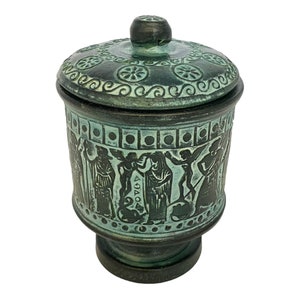The photograph showcases a close-up image of an antique urn, placed against a pure white background. The urn appears to be quite old and is made out of metal, likely copper, given its oxidized dark green to almost black color with spots of faded green. Its design is cylindrical, comprising a tapered base, a wider cylindrical body adorned with intricate engravings, and a removable lid that curves slightly downward with a knob at the center. The carvings feature figures resembling Egyptian deities or possibly ancient Roman, Greek, or even angelic figures, including people in robes and symbols that add to its historical aura. The image is clear, well-lit, and devoid of any other objects, emphasizing the urn's detailed engravings and aged patina.